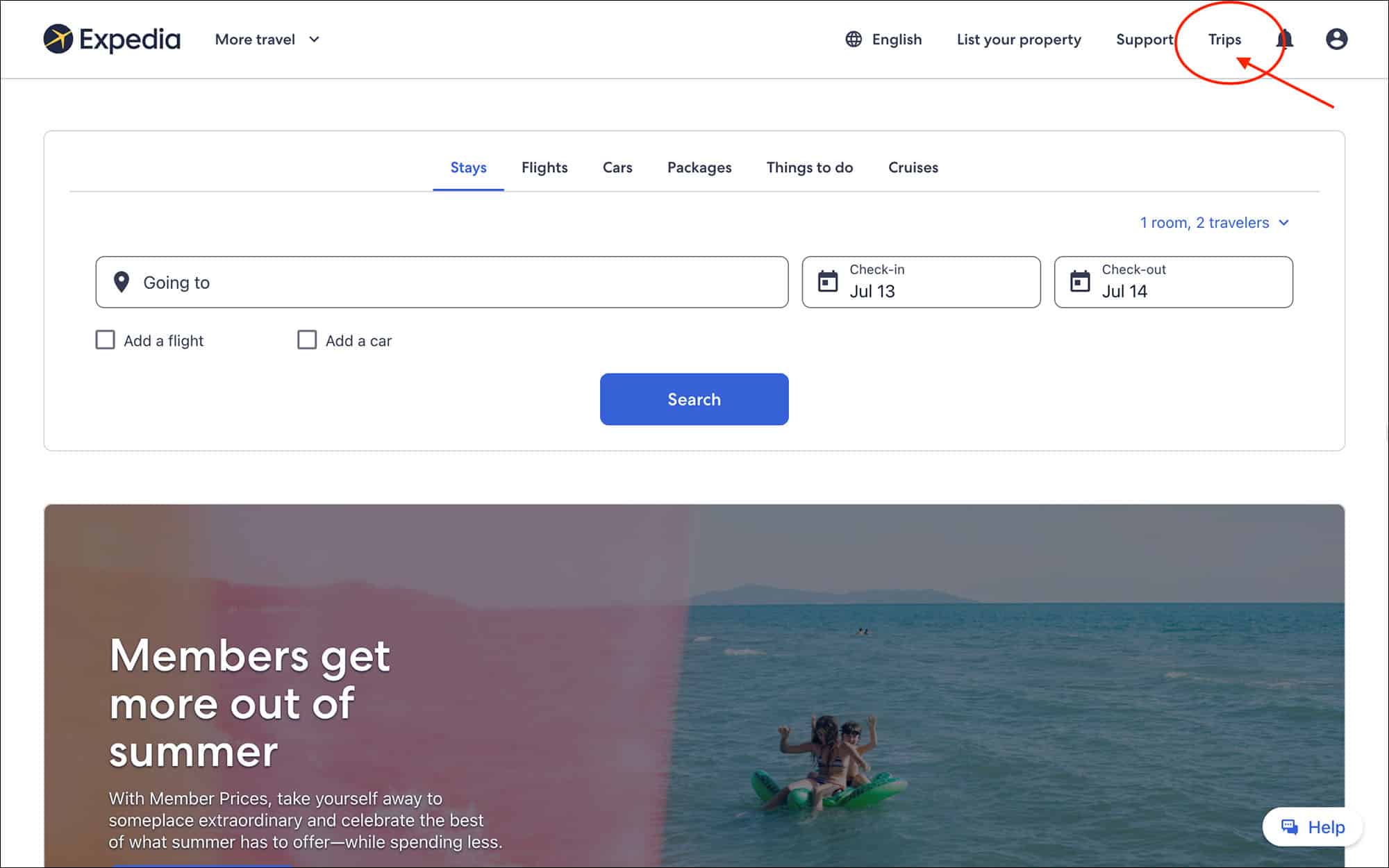The image depicts a webpage from Expedia, characterized by various interface elements and promotional content. 

In the top-left corner, the Expedia logo is visible, featuring a blue circle with a yellow shape resembling an airplane. Immediately to the right of the logo is the phrase "More Travel" accompanied by a downward-pointing arrow. 

On the top-right, the page displays multiple options: "English" is listed next to a globe icon; following this are "List Your Property," "Support," and "Trips." The "Trips" option is notably highlighted with a red circle and an inward-pointing red arrow. Adjacent to these options are a bell icon and a profile icon.

Below this navigation bar, there is a series of tabs labeled "Stays," "Flights," "Cars," "Packages," "Things to Do," and "Cruises," with the "Stays" tab highlighted in blue. Beneath these tabs are several interactive fields. The first field is labeled "Going To" and includes a location icon. To its right, there are fields designated for "Check In" and "Check Out," with dates set to July 13th and July 14th, respectively. Above these fields, it indicates "One Room, Two Travelers" in blue text. 

Additionally, there are two checkboxes below these fields labeled "Add a Flight" and "Add a Car," both currently unchecked. The "Search" button is prominently displayed in blue beneath the checkboxes.

Further down, a promotional section reads, "Members get more out of summer." This section describes the benefits of member prizes, encouraging users to "take yourself away to someplace extraordinary and celebrate the best of what summer has to offer, while spending less." Accompanying this text is an image of two children joyfully riding a green flotation device in the ocean.